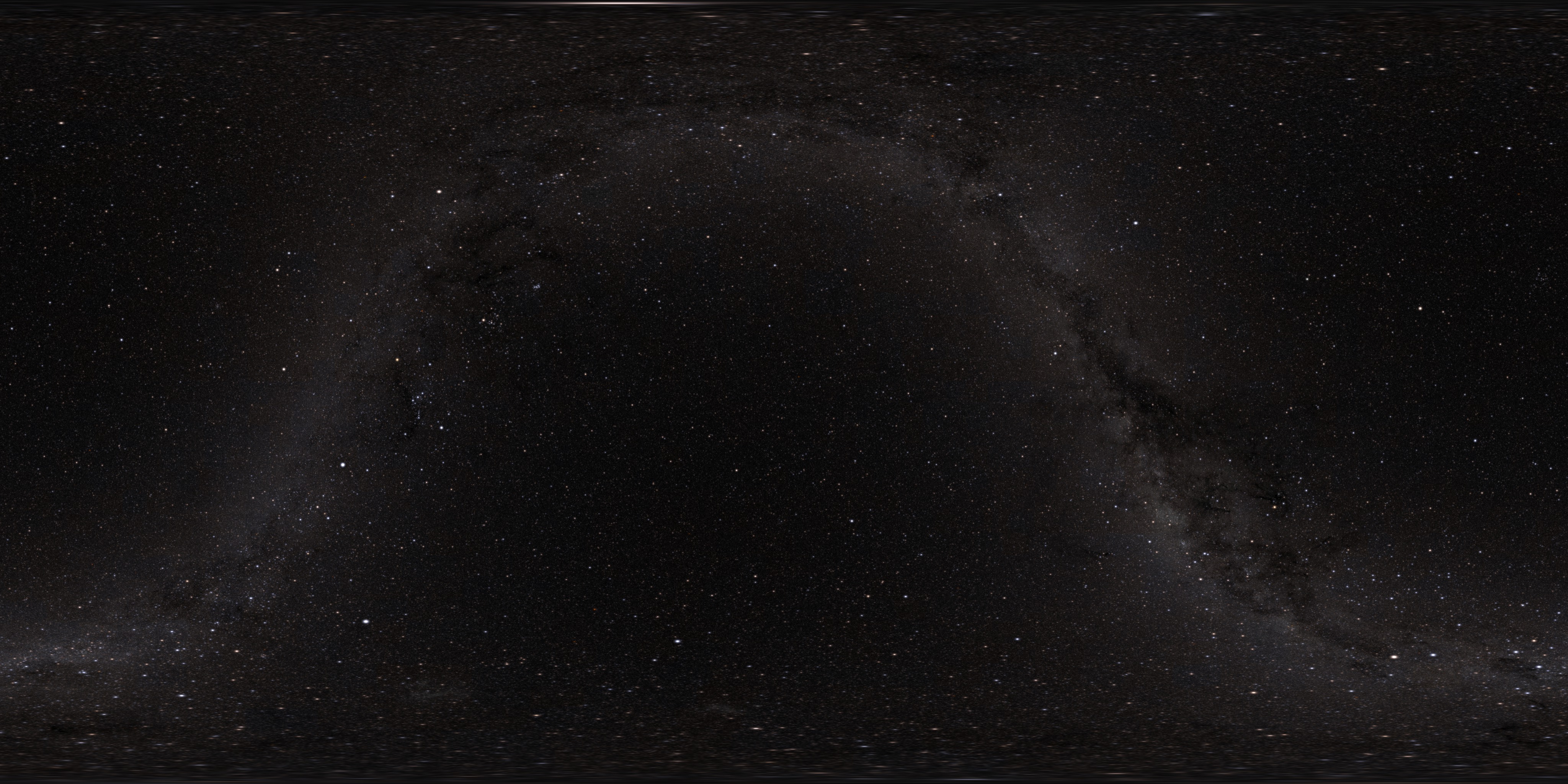This photograph, taken at night with likely the aid of a telescope, captures an inky black sky teeming with numerous, sharply defined stars. The image is rectangular and predominantly dark, though various stars are scattered across the middle, left, and right sections, appearing as small white dots. A distinct feature in the center of the photograph is an area where the stars and possibly a faint white mist or haze form a notable "hump" or hillock shape. This feature starts at the bottom left, arcs upward and curves downwards, creating a dome-like plateau that stands out against the black sky. The stars in this region are densely clustered, suggesting a possible constellation. The photograph is devoid of any planets or spacecraft, presenting a pure and unobstructed view of the night sky, with galaxies and stars enshrouded in minute areas of dark space. The overall composition, with its clear depiction of cosmic details and the hillock-like formation, conveys a serene and expansive celestial landscape.